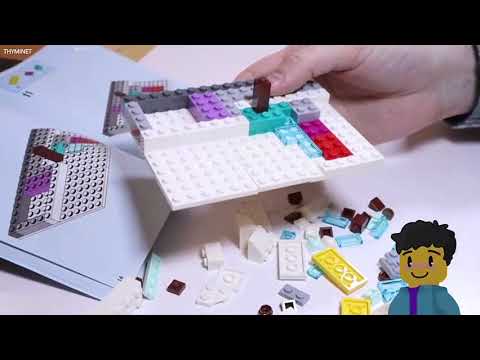The photograph showcases a detailed scene of a person intently working on a Lego set. Only their right hand is visible, emerging from the right side of the frame, holding an assembled piece of the set. The piece comprises a flat white base with a variety of attached blocks in colors like gray, light gray, light blue, red, transparent blue, and other hues such as teal, purple, pink, and orange. The setup is on a white tabletop covered with a spread of additional Lego pieces in shades of yellow, white, and gray. To the left, an open instruction book reveals a page that matches what the hand is constructing, indicating ongoing progress. The top left corner of the image features the text "The Mitt," while the bottom right corner includes a cartoonish illustration of a Lego character with black hair, dressed in a blue cover over a purple shirt, peering above the black border. Both the top and bottom of the photograph are framed with half-inch black bars.